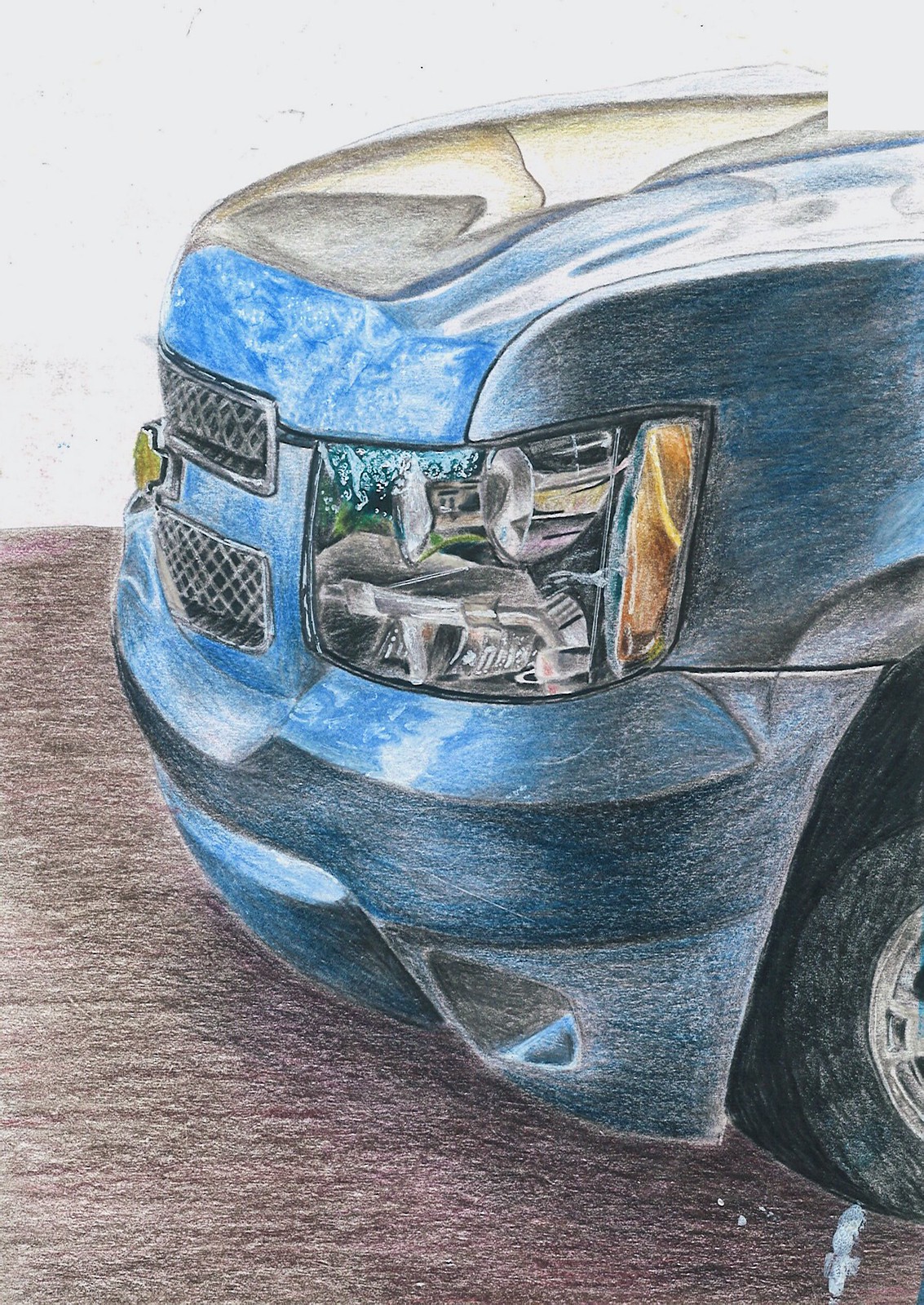This is a detailed color pencil drawing of the front end of a blue Chevrolet vehicle, likely a van or an SUV, captured from a left-side angle. The artist has meticulously rendered the front bumper, grille, and left headlight, showcasing impressive attention to detail. The headlight is intricately drawn with visible reflections and inner workings, including various metal tubes and a yellow cylinder. The shading employs a range of blues, grays, and blacks to emphasize the metallic texture and reflections. The ground beneath the vehicle is illustrated in a dark brown, resembling a dirt road, while the background remains plain white, giving the drawing a stark contrast. Despite some amateur qualities, the piece exhibits considerable effort and skill in its color and shading work, although it lacks a signature.